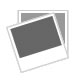This close-up photograph showcases a slender black belt crafted from a material mimicking faux alligator or snakeskin, characterized by its small, intricate scales. The belt is arranged in a circle within the image, with its end tucked on the inside and the buckle on the outside, at the bottom. The belt's surface has a silver sheen, contributing to its detailed look. It features a pewter-colored buckle with a subtle, swirly design and a metal clip for securing the belt. The reverse side reveals a tan suede-like texture, contrasting with the black faux leather exterior. The background is simple, formed by a white floor and wall, emphasizing the belt as a fashion piece on display. Multiple holes can be seen along the belt, highlighting its functional design.